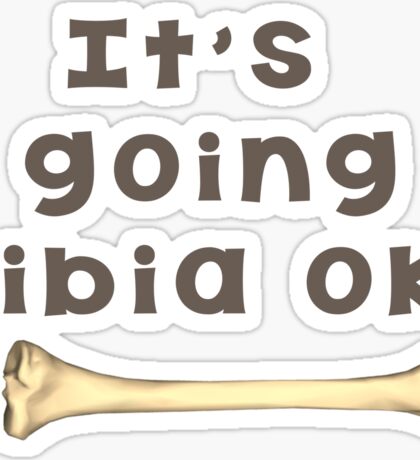This image is a digital creation, likely designed for sharing as a humorous meme on social media. Dominating the top 90% of the image is text in a whimsical, dark gray font that reads, "It's going tibia okay," although the words are partially cut off, creating a playful distortion. The text is encircled by a fluffy, cloud-like outline in white, further bordered by gray. The background is a subtle pale gray, adding to the modern, illustrative feel of the scene. Positioned at the very bottom of the image and spanning its entire width is a horizontally aligned tibia bone, rendered in cream tones with light beige and gray highlights, contributing to the overall whimsical style.